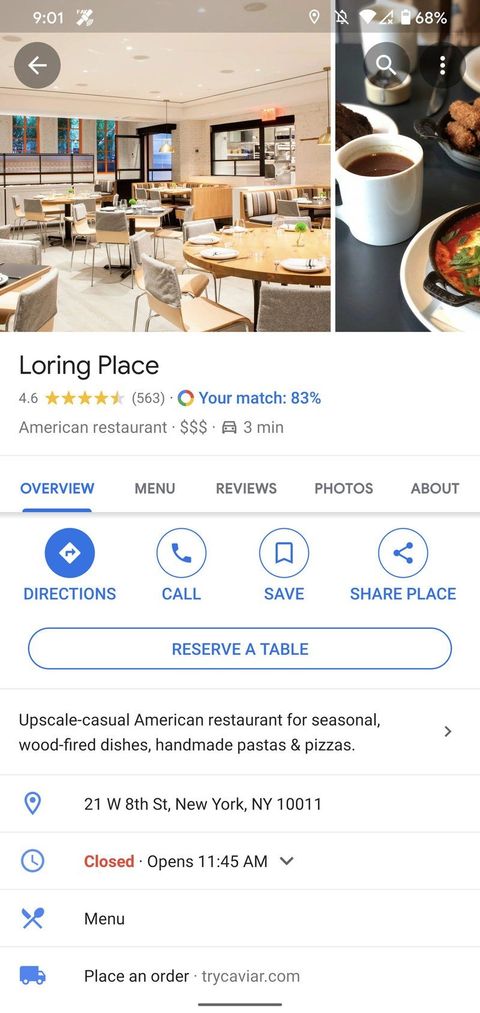This image is a detailed screenshot of a Google business page for a restaurant named "Loring Place." At the top of the page, there are photos showcasing the restaurant's interior, featuring a modern dining room with circular wooden tables and white chairs. Beneath the photos, the business name "Loring Place" is prominently displayed, followed by its rating of 4.6 out of 5 stars, based on 563 reviews. It also shows a personal match score of "83%" highlighted in blue.

Further details identify Loring Place as an "American restaurant" with a price range denoted by three dollar signs, indicating a moderately expensive dining experience. A stopwatch icon indicates that the restaurant is located 3 minutes away. 

Directly below this information, there are five navigation tabs: Overview (which is underlined and highlighted in blue), Menu, Reviews, Photos, and About. Additionally, the page features four circular action buttons—Directions, Call, Save, and Share Place—each with blue icons in their centers.